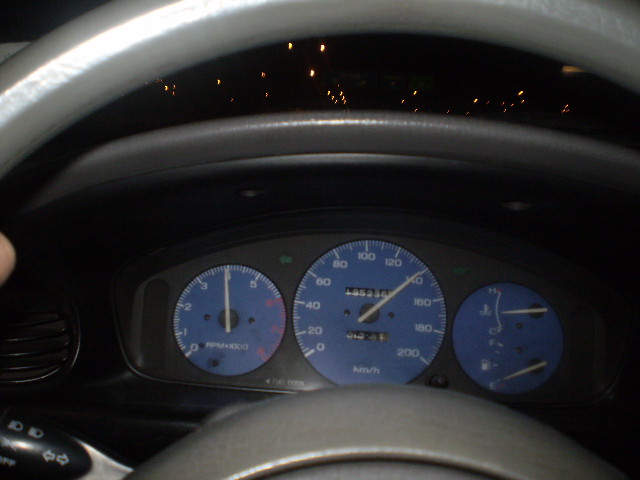In this nighttime photograph taken inside a vehicle, the dashboard displays various indicator dials, including gauges for fuel and speed. On the left edge of the image, a barely visible finger is grasping the steering wheel, suggesting the driver is either in motion or parked. The background, visible through the windshield, is pitch black, hinting at nighttime driving conditions or the possibility of being in a low-lit parking lot. The dashboard area features a two-tone gray interior, with the dial faces illuminated in blue and marked with white numbers and hands. The exact status of the vehicle's movement remains indeterminate, adding an element of mystery to the scene.